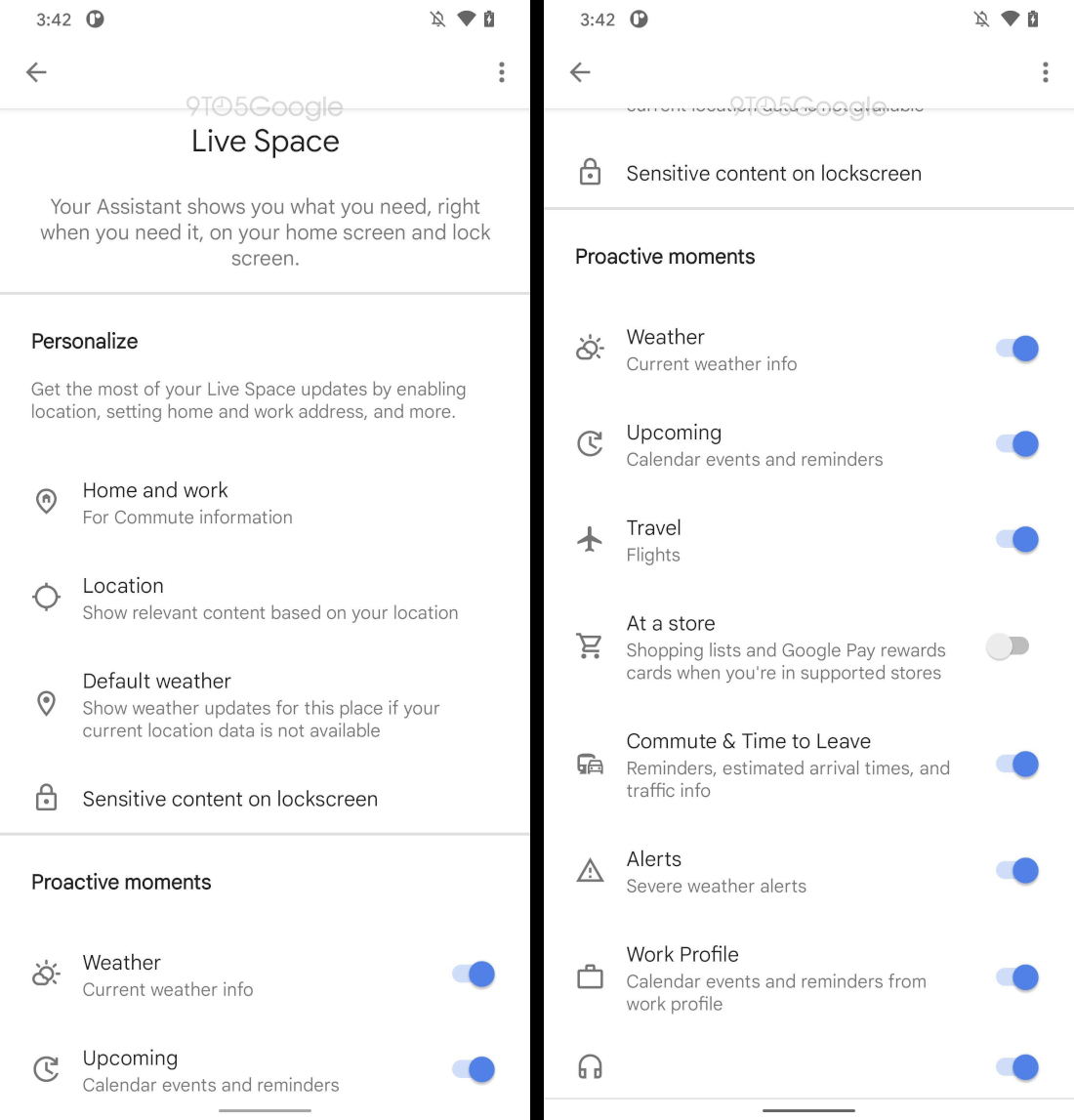The image consists of two side-by-side screenshots divided by a black vertical bar. Both screenshots feature a predominantly white background, and display identical elements at the top: a time stamp "3:42" in the top-left corner, a black circle with a white "P" inside it, a right-aligned battery icon, full Wi-Fi signal indicator, and a muted sound icon. Additionally, there's a black arrow on the left side of each screenshot.

Centered in gray text, both screenshots read "9T05 Google," followed by "Live Space" in a larger font. Beneath that, the text reads: "Your assistant shows you what you might need right when you need it on the home screen. I'll lock the screen." Below this section is a thin gray border.

In the first screenshot, black text labelled "Personalized" appears along with two lines of descriptive information. Below this, on the left side, four icons are listed with their corresponding names and functions. This is followed by a thin gray line and another section labeled "Proactive moments," which includes two more icons accompanied by descriptions and toggles, both of which are turned on.

The second screenshot is similar but features different content below "9T05 Google." The line under "Live Space" reads: "Sensitive content on lock screen" and is underlined, followed by another "Proactive moments" section. This screenshot appears to have been scrolled down further, displaying eight more icons along the left side, each with corresponding names and information. On the right, the top three toggles are highlighted in blue (indicating they are on), the fourth is in grey (off), and the remaining four are also blue (on).